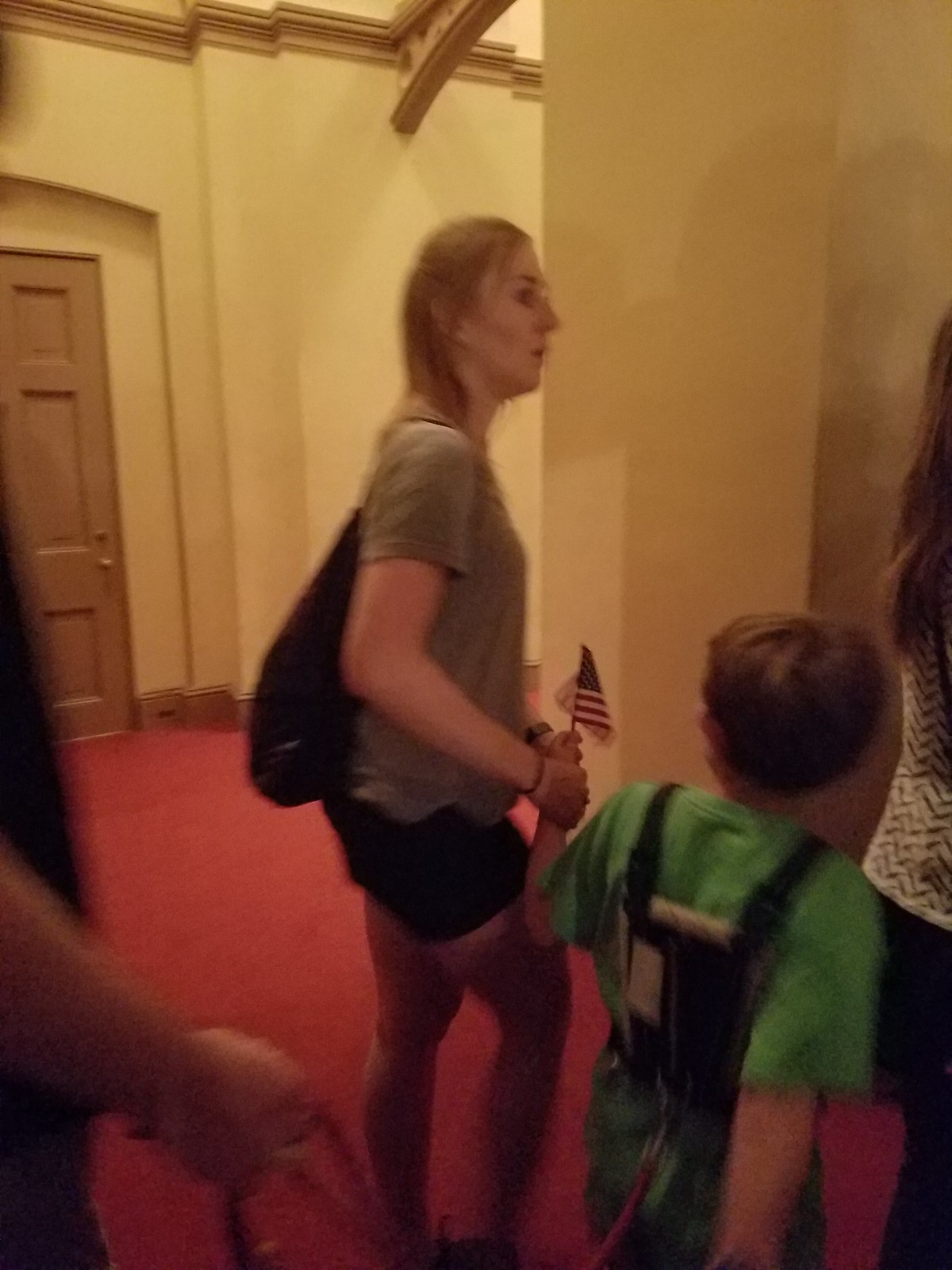In this slightly blurry, low-quality, portrait-style image, we see a scene likely captured in a hall or possibly a church. The background features yellow walls and a light brown door to the left, with an orange-reddish carpet covering the floor. Central to the image is a blonde-haired woman in her 30s, wearing a grey t-shirt, black knapsack, and blue shorts. She is holding the hand of a young boy, who has dark hair and is wearing a green shirt and a black and red harness. The boy, holding a small American flag in his hand, appears to be connected to another person behind him wearing a black t-shirt, who holds the harness's string. Another woman with long brown hair, dressed in a white and black top and possibly a black skirt, stands in front of the boy. The scene appears to show a group of people lined up, with only portions of some figures visible, adding to the image's overall enigmatic feel.